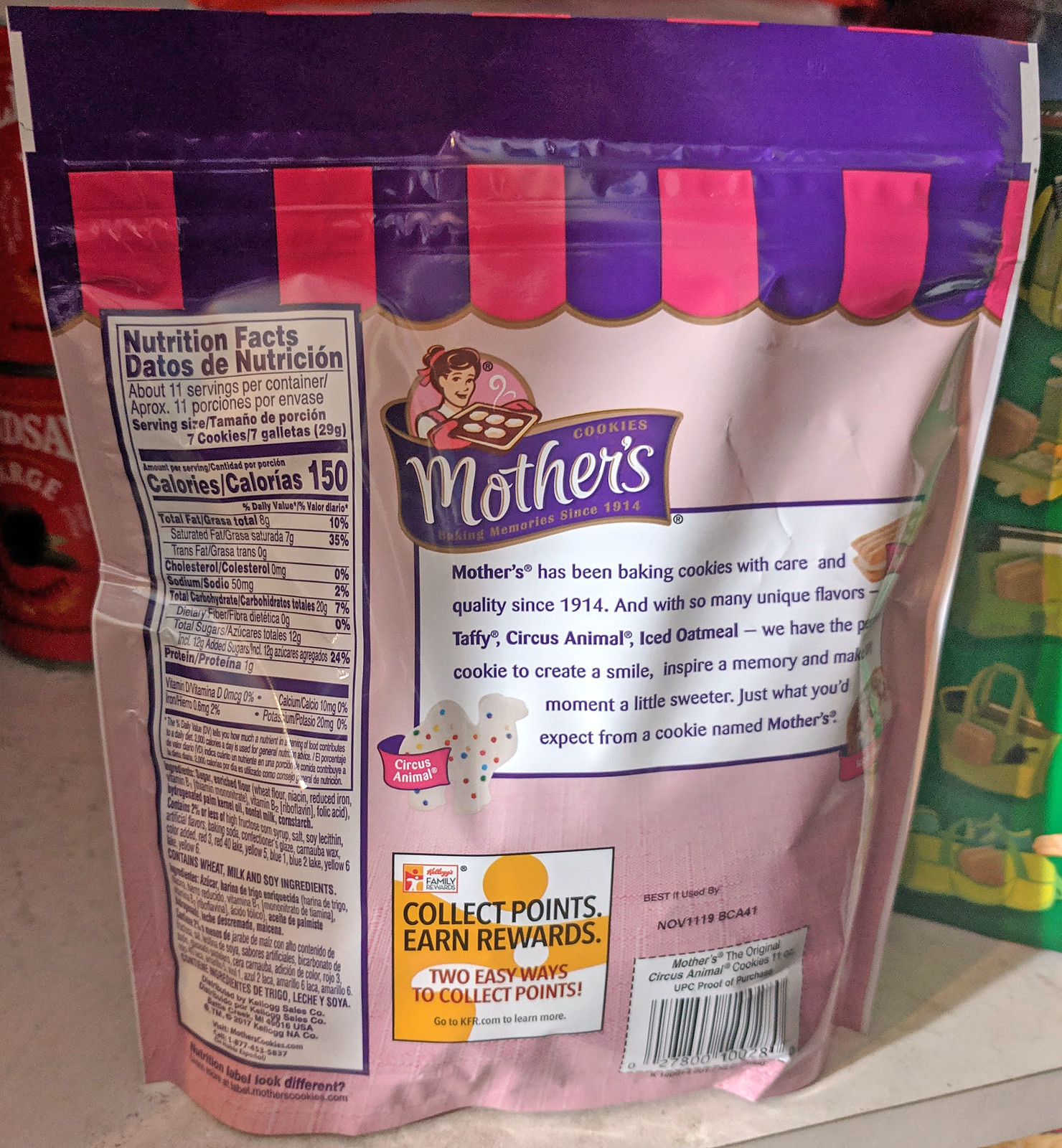The image features the back of a bag of Mother's Cookies, prominently displayed in a mostly light purple plastic packaging. The top of the bag, where it can be torn open, alternates between purple and red sections. Centrally located is a vertical white box containing nutritional information, which includes details such as calories and other dietary data. 

To the right of the nutrition facts box, there's the Mother's Cookies logo – a purple emblem resembling a flag with white lettering. This logo also includes a vintage-styled illustration of a woman holding a tray of freshly baked cookies. 

Towards the bottom of the bag, there is an orange and white box that reads "Collect Points, Earn Rewards." Additionally, the bottom-right corner features a small box containing a barcode. The bag is placed on a white table, with a green object partially visible behind it on the right side, and a red item, potentially a coffee cup, on the left side.